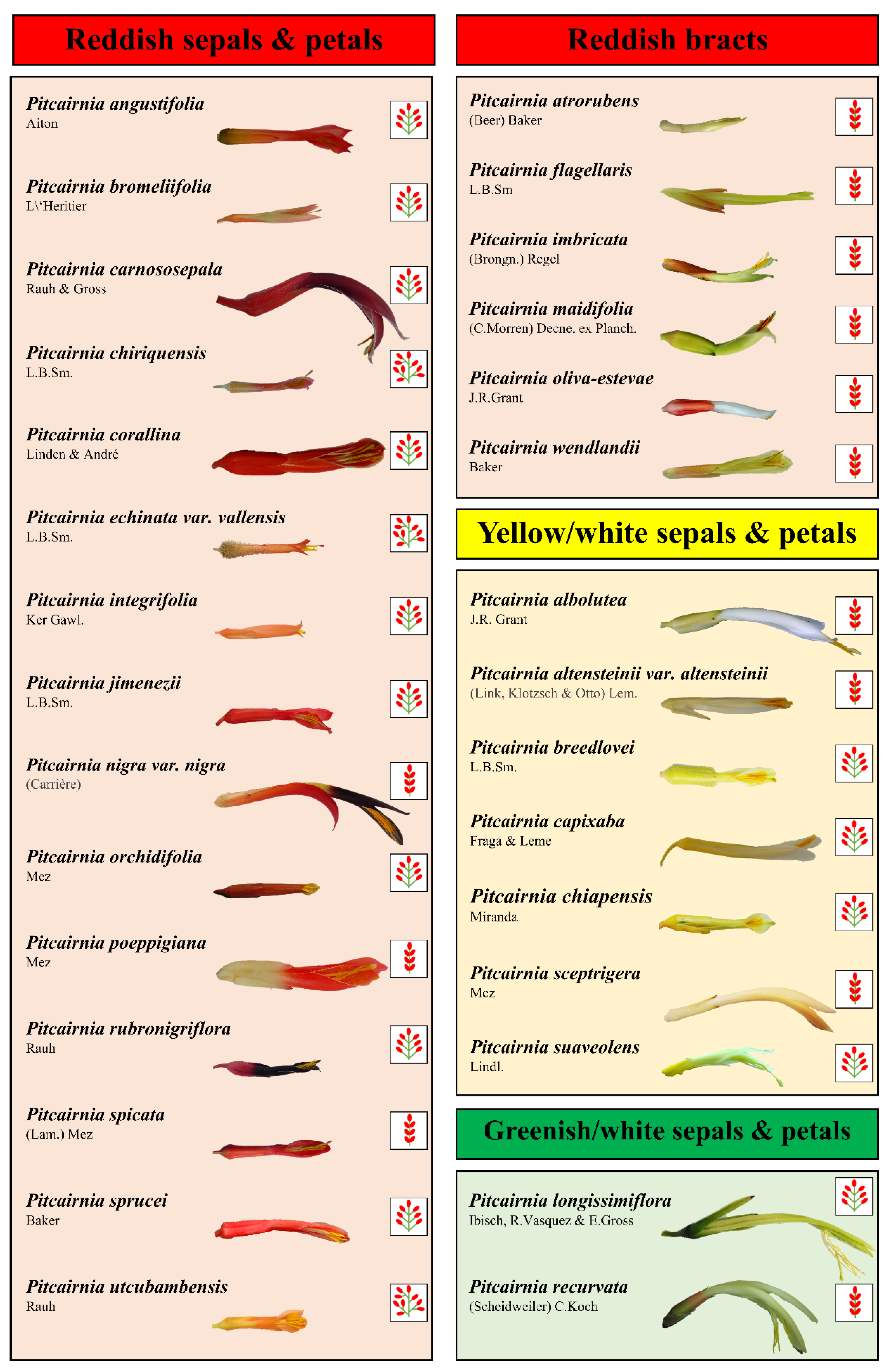This comprehensive infographic visually categorizes various floral species based on the color of their sepals and petals. The image is divided into several distinct sections, with each section dedicated to a specific color category:

- **Left Side (Vertical Section):** Occupying the entire left half of the image, this vertical rectangle features a red header labeled "Reddish Sepals and Petals." Beneath this header, a light pink background showcases a detailed list of around 10 to 15 species. Each entry includes the scientific name of the species alongside a corresponding image depicting the flower in full bloom.

- **Right Side (Three Vertical Sections, Top to Bottom):**
  - The **top section** mirrors the left in design, with a red header stating "Reddish Bracts." Below this header, set against a red background, are six scientific names accompanied by images of the respective species.
  - The **middle section** focuses on species with "Yellow/White Sepals and Petals," indicated by a yellow header. This section, against a light yellow or cream background, contains around seven species' names and their corresponding images.
  - The **bottom section** features a green header labeled "Greenish/White Sepals and Petals." This smaller section, set against a light gray background, lists two species along with images of each.

Overall, the infographic provides a visually organized and detailed guide to identifying various species by the color of their sepals and petals, complete with scientific names and illustrative images.